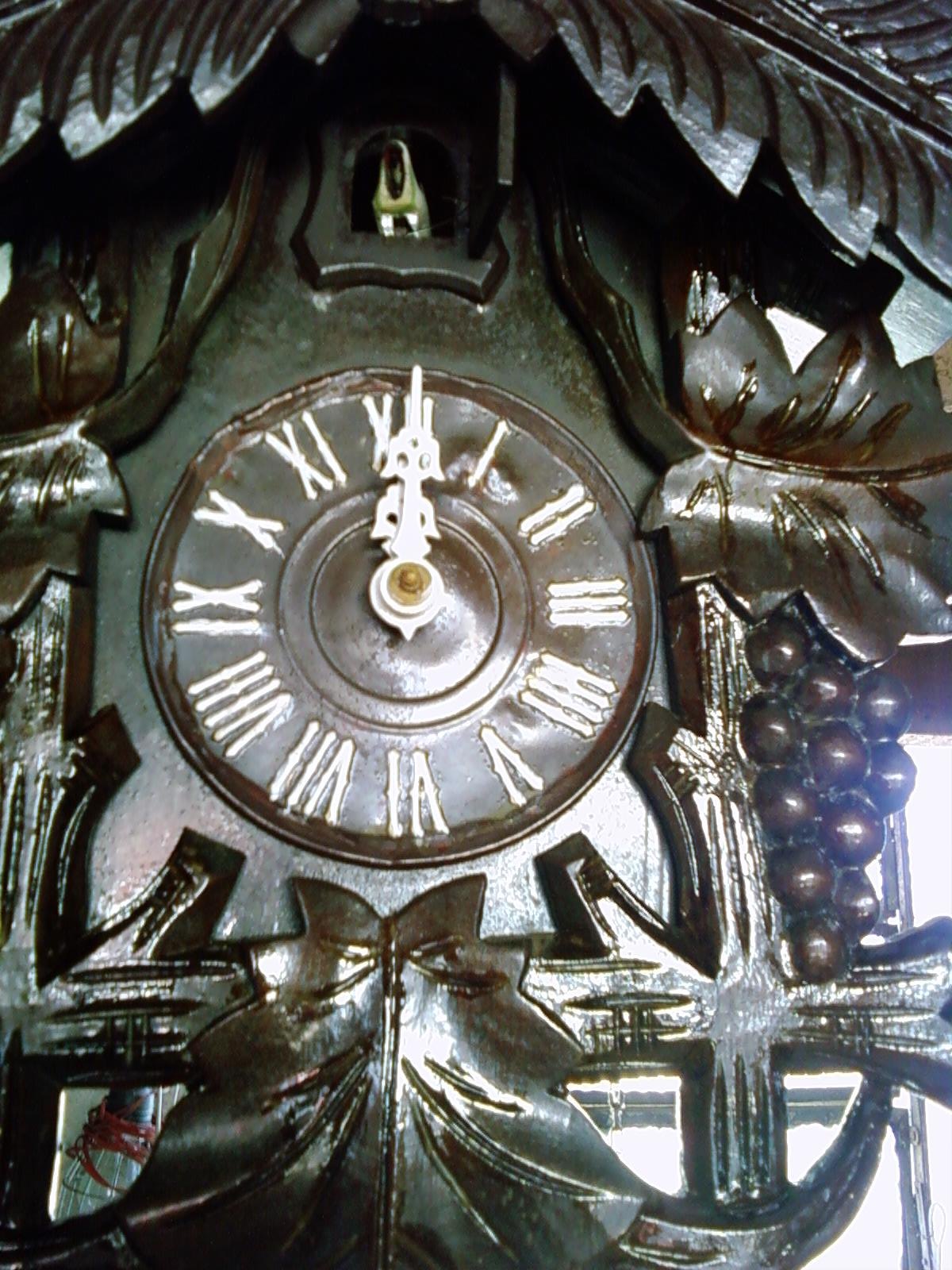The image features an ornate antique grandfather clock made primarily of brass. This exquisite timepiece boasts an intricate design, adorned with large brass leaves and vines of grapes intricately woven into the frame, adding a touch of elegance and vintage charm. At the top of the clock, a small window suggests a functional feature, likely used for a cuckoo mechanism that activates when the clock strikes twelve, potentially revealing a small bird or figure. The clock face is classical and sophisticated, displaying Roman numerals from I to XII instead of standard numbers, further enhancing its timeless appeal.